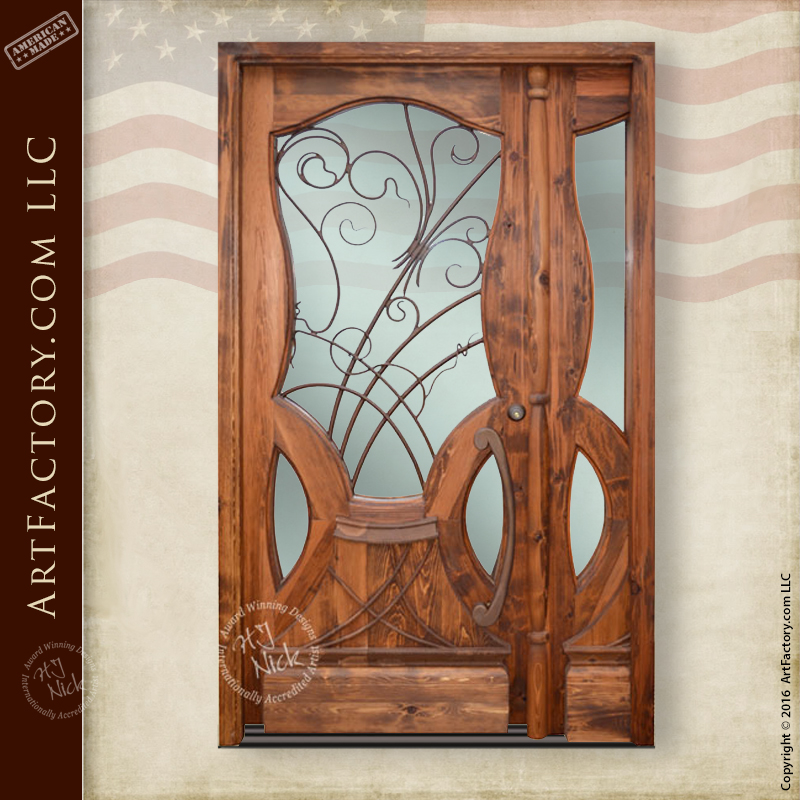The image depicts an ornate wooden door with intricate glass paneling featuring decorative metal vines and curves, suggesting an air of craftsmanship and artistry. The door, a rich brown with a visible handle and lock, is the central focus against a backdrop that blends an old paper texture with a tan version of the American flag. On the left side of the image, a dark brown strip runs vertically, inscribed in all-caps yellow font with "Artfactory.com LLC" and a logo labeled "American Made" adorned with four stars. The image also includes multiple watermarks and text including "Award-winning designs, internationally accredited artist H.J. Nick" and "Copyright 2016 artfactory.com LLC." This image is part of a Western States project and will be shared with a broader team at a later time.